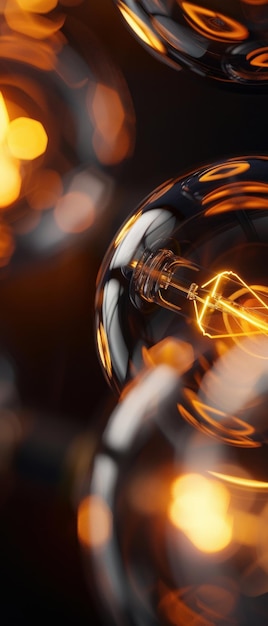The image shows a close-up view of an incandescent light bulb within a mechanical process, possibly depicting its interior. The photograph, rectangular in shape, focuses on a filament that emits a dim, warm glow, casting hues of gold, amber, and mid-tones of brown against a predominantly amber backdrop. The glass bulb appears smoky brown and reflects various illuminated elements. The bulb is prominent in the foreground but not fully in frame, extending from the right side towards the left. Additional blurred light sources, likely other bulbs, create flecks of orange on the left and bottom right against a dark background. The entire setting is enveloped in deep browns, with several curved edges suggesting multiple bulbs in the fixture. The detailed composition captures the complexity and subtle variations in light and shadow within the image.